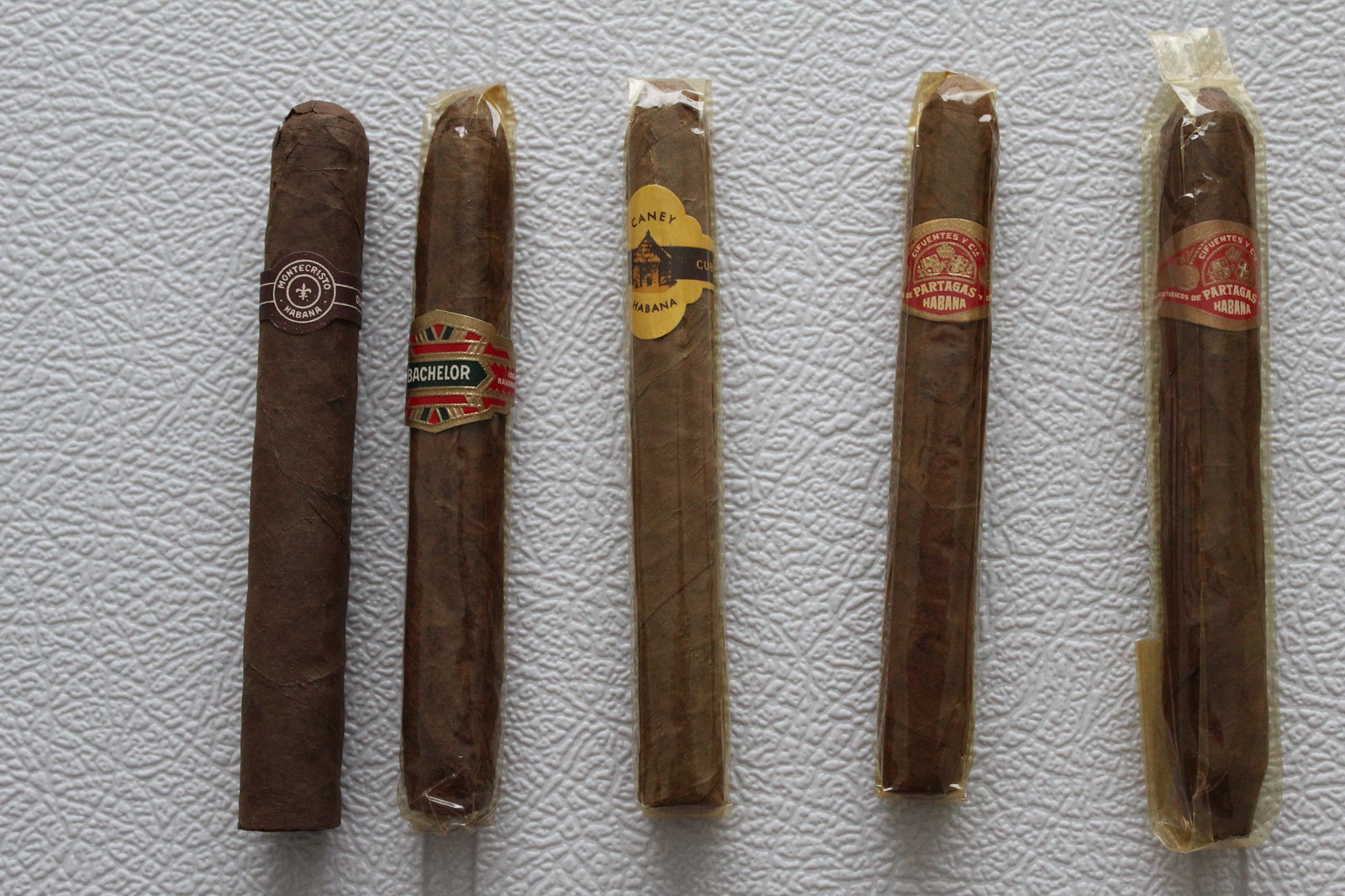The photograph, which is rectangular and wider than it is tall, displays five Cuban cigars meticulously arranged in a row on a textured white vinyl surface. The leftmost cigar, unwrapped and ready to smoke, features a brown label with white lettering that reads "Monte Cristo Habana," adorned with a fleur-de-lis emblem. Moving right, the second cigar, encased in yellowing plastic, boasts a green, gold, and red label with the word "Bachelor" in white letters set against a decorative background. The third cigar, slightly thinner and lighter, showcases a yellow label with a house emblem and the words "Caney Habana." The final two cigars, both wrapped in clear plastic, have identical red and gold embossed labels reading "Partagas Habana." The cigars' earthy brown casings contrast subtly against the white, rugged vinyl, highlighting their intricate packaging and suggesting a hand-rolled craftsmanship.